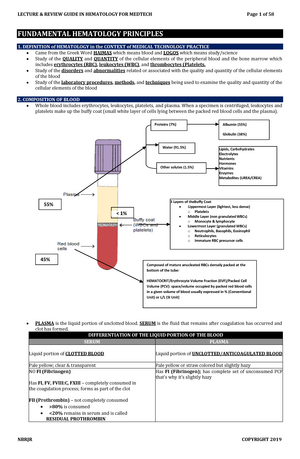The image depicts a detailed page from a science textbook or lecture guide focused on hematology. Centered at the top, the title prominently reads "Fundamental Hematological Principles" in bold lettering, set within a black bar. Below the title, there's a subheader with bullet points summarizing key concepts. The layout includes a diagram showcasing a blood collection vial, which has a purple cap and contains a beige solution representing plasma, with red denoting the blood sample. Surrounding this central diagram are various tables and dense text, providing extensive information relevant to blood testing and hematological procedures. The text and diagrams are in black, white, red, light purple, light yellow, and gray, set against a solid white background.